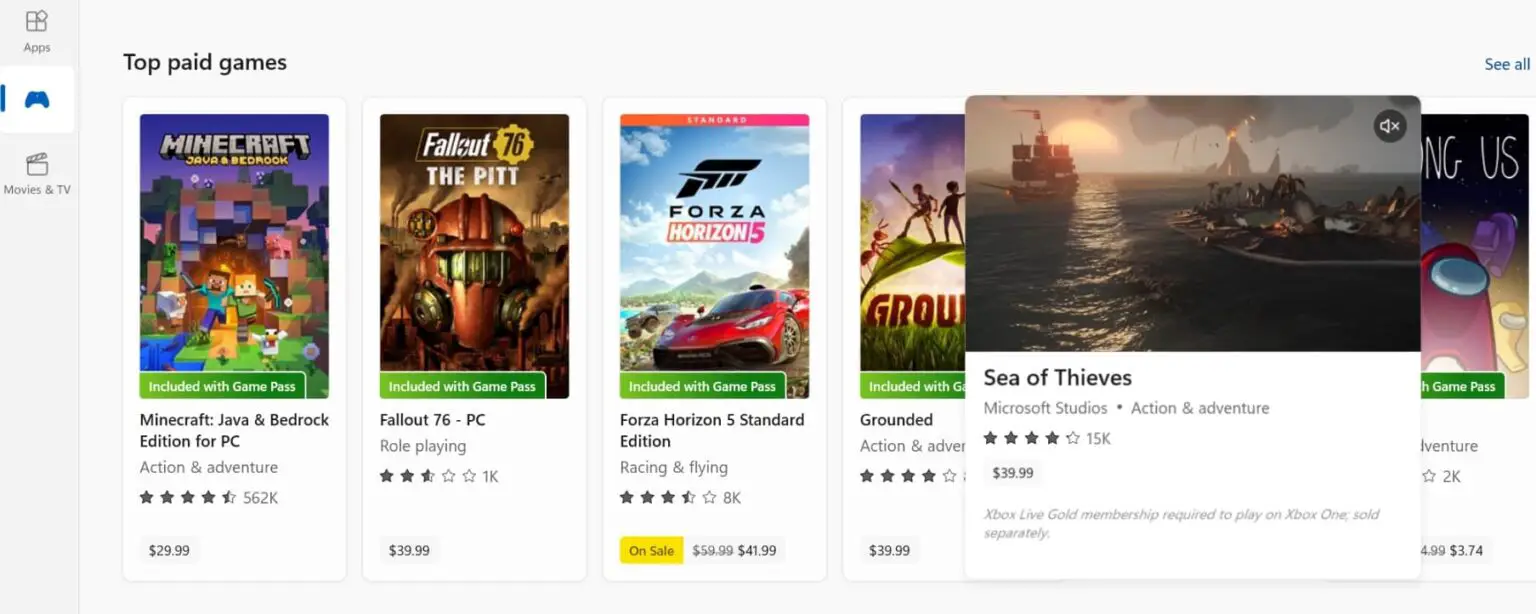In this screenshot of a game seller's webpage, the header prominently features the black text "Top Paid Games" against a white background. Below this heading, various game covers are displayed, including Minecraft, Fallout: The Pitt, and Forza. Dominating the center of the image, a significantly larger and selected game cover for "Sea of Thieves" obscures the last two game titles. On the left side of the page, three vertical logos labeled "Apps," "Games," and "Movies & TV" are displayed, with "Games" currently highlighted. In the upper right corner of the page, the option to "See All" is available in blue text.